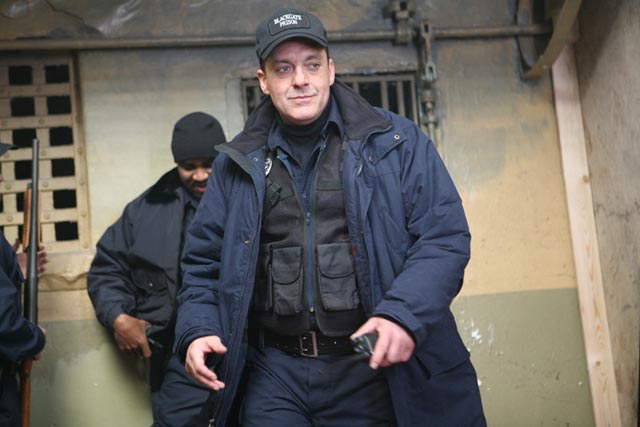In the center of the image, there is a man wearing a dark black cap with white lettering, which partially obscures his face as he looks to the right. This man, seemingly a policeman, is mid-stride, clad in a long dark blue coat over a black vest that has multiple pockets. Underneath the vest, he wears a dark blue collared shirt and a black turtleneck, paired with dark blue pants and a black belt featuring a silver buckle. In his left hand, he carries a black object, possibly a radio or taser, and his arms are positioned slightly in front of him. 

To his left, partially visible, is another person holding a rifle with a black barrel and a brown stock. Behind the central figure and slightly to the left stands another man wearing a black woolen cap, dark blue jacket, and dark blue pants. This second man, an African American, is looking down with his hand resting on a gun. The backdrop of the image is a wall made of either cinder block or plaster, featuring barred windows.